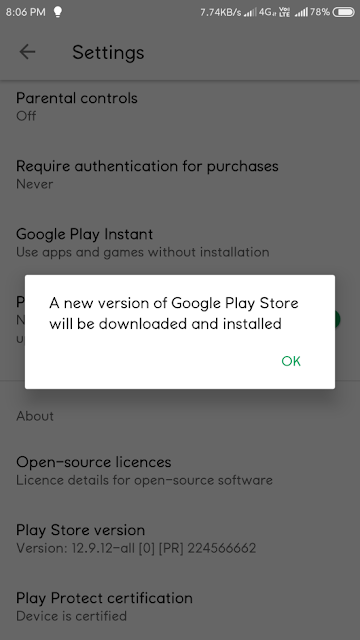The image captures a screenshot of the settings on a Google Android phone, specifically within the Google Play Store app. The current screen displays various settings including "Parental Controls: Off," "Require Authentication for Purchases," and the app version, listed as 12.9.12. 

In the midst of navigating these settings, a pop-up notification appears, dominating the screen. This notification, presented on a white background with black text and a green "OK" button, informs the user that a newer version of the Google Play Store is available for download and installation. The message disrupts the user experience, emphasizing the need to update the app for continued use and access to the latest features. The background of the screenshot still shows the preceding settings screen, partially obscured by the update prompt.